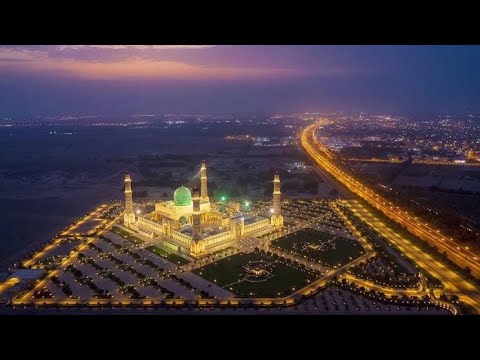The image captures a vibrant nighttime cityscape, dominated by a majestic structure reminiscent of a mosque or palace, bathed in thousands of yellow lights. This central structure features a prominent green dome and is flanked by four towering minarets at each corner, with walls and intricate lighting patterns creating a striking visual. The mosque or palace is enclosed in an elaborately lit square with a mix of green and yellow lights, enhancing its grandeur.

To the right of this lit square, an orange-lit highway curves gracefully into the distance, merging with a sprawling cityscape of twinkling lights. This highway, lined with street lamps, appears to be an interstate or a large four-lane road, bustling with illumination as it stretches towards the horizon. Skirting the left side of the highway is what seems to be a parking lot, transitioning into a courtyard or landscaped area filled with grass and possibly fountains or monuments.

The night sky above is adorned with an orangish-pink hue from the setting sun, blending into deep purples, making the city glow even more brilliantly. The entire scene is reminiscent of a festive display or the view one might encounter while approaching a bustling city at night, with countless lights creating a magical, almost dreamlike ambiance. A black stripe across the top and bottom of the image frames this intricate panorama, emphasizing the landscape's rich and vibrant details.